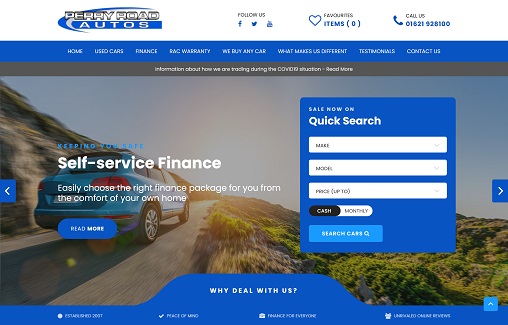On the main page of an automobile company's website, a detailed and intricate logo is prominently displayed at the top in silver and white hues. The exact address is somewhat unclear, suggesting either "Derry Road" or "Perry Road." On the left side, the company name "Otto's" is listed. To the right, there are prompts to follow the brand on social media platforms such as Twitter and Facebook.

Below the logo area, a navigation bar is displayed with a blue banner leading to the home page and various other sections, followed by another gray banner with text that is difficult to read due to its small white font. The focal point of the page features a striking image of an automobile viewed from behind, cruising along a desolate single-lane road into the sunset. Superimposed on the image is a call to action in white text that reads "Self-serve finance," with an indecipherable blue text above it.

Further down, the caption "Easily choose the right finance package for you from the comfort of your own home" is provided, along with a clickable link for more information. To the right, there's a quick search function where users can input their details if they know exactly what they are seeking.

Additionally, the front page includes navigation options allowing users to click left or right to discover reasons for dealing with the company, emphasizing that the auto company is keen on encouraging purchases from their platform.